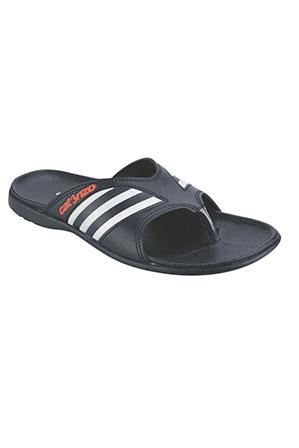The image showcases a high-quality, black leather sandal designed for men, likely intended for casual or sports use. Set against a blank white background, the sandal features a low cut and low heel, with an open back for easy slip-on comfort. The front of the sandal is flat, while the slightly cushioned back offers about a quarter inch of height. A unique three-stripe design in black and white adorns the sides, and the brand name, indicated by the red lettering "CATNZO," is partially visible. The sandal includes a separation for the big toe and has a pointy, V-shaped front, reminiscent of a Batman-like design, enhancing its distinctive look. The robust build and waterproof material, along with traction grips on the bottom, further emphasize its practical, everyday wear capabilities.